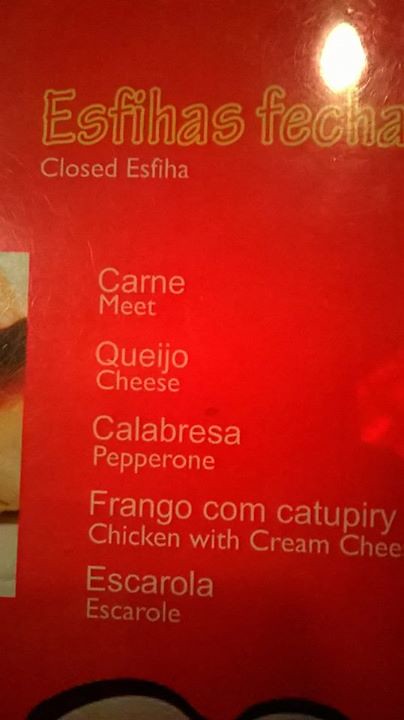The image is a color photograph of an illuminated plastic or acrylic sign displayed in a restaurant. The sign is backlit, glowing intensely, and additional light reflecting off the top right adds to its brightness, resembling the effect of looking into the sun. This stray light appears to come from a fixture behind the viewer.

The main portion of the sign is red, with the left side showing a sliver of a cropped photo illustration, leaving the content of the illustration indiscernible. The top of the sign features the text "Esfihas Fecha" in yellow outlined letters, although "Fecha" is incomplete and might continue off-frame, potentially intended to be "Fechada." The language used appears to be Portuguese, not Spanish, given the spelling and phrasing.

Below this title, the sign lists various food items with their English translations:
1. "Esfihas" translates to "closed" in white letters.
2. "Carne" is intended to mean "meat" but is misspelled as "MEET."
3. "Queijo" translates correctly to "cheese."
4. "Calabresa," meaning "pepperoni," is misspelled with an extra 'E' at the end as "PEPPERONIE."
5. "Frango com Catupiry" translates to "chicken with cream cheese," though it's noted as "chi" before being cut off, suggesting the full word "cheese."
6. "Escarola" translates to "escarole."

The bottom of the sign features a thick wavy brushstroke design, indicating it may be the upper portion of a larger illustration that is cropped out of the photograph's frame.